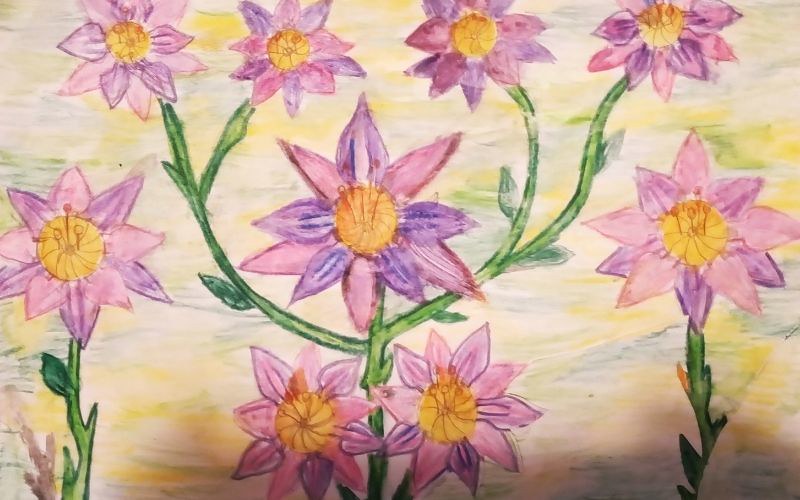This image depicts a serene and artistic representation of flowers, evoking the delicate style of watercolor or possibly colored pencils. The background merges soft hues of yellow, white, and hints of gray and green, enhancing the tranquil ambiance. Central to the image is a green stem that branches into multiple vines, each adorned with flowers featuring purple and pink petals with yellow or orange centers. Flanking this central arrangement are two singular flowers on either side, each showcasing thicker green stems and leaves, with distinctive flowers characterized by pink and purple petals and orange centers, some accented with small red lines and dots. The composition includes pairs of flowers strategically placed beneath the central cluster, contributing to the overall harmony and complexity of the image. The details and colors used in the flowers suggest a meticulous and thoughtful artistic approach, underscoring the peaceful and picturesque quality of the scene.